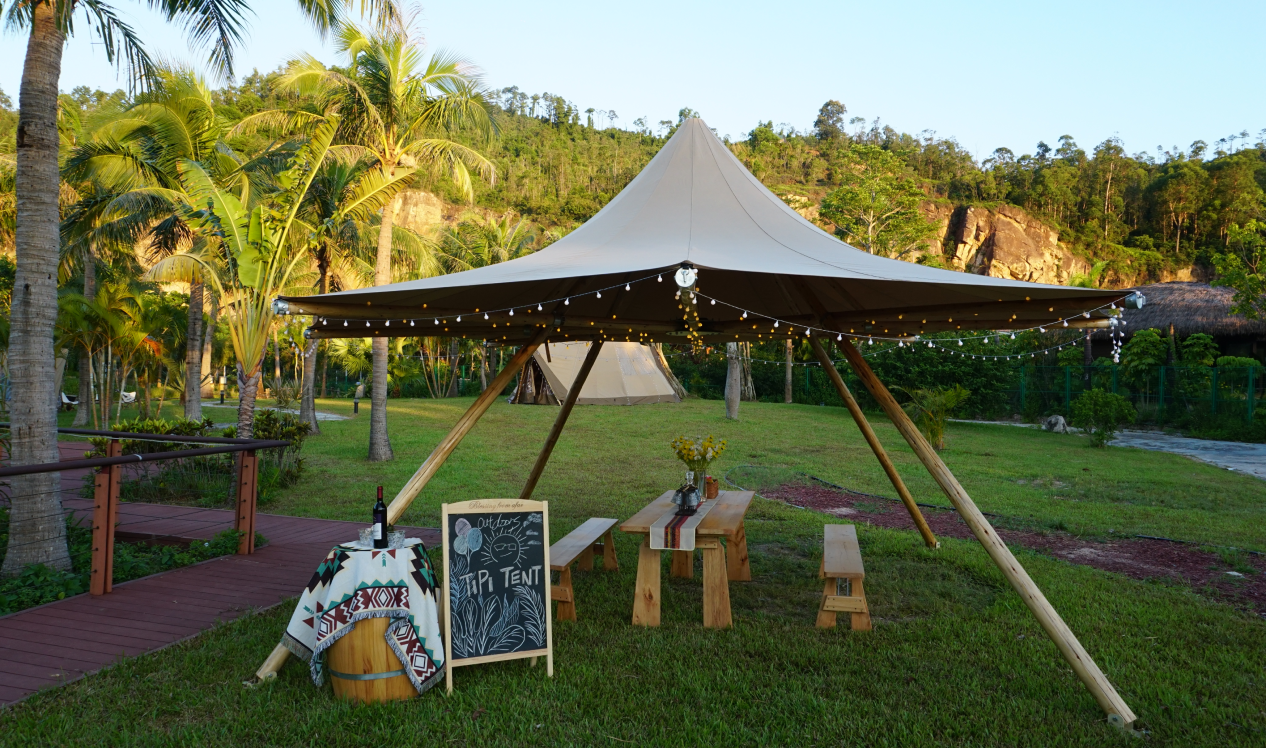The photograph captures a serene, green outdoor setting, either a backyard or a park, illuminated by a clear sky. The scene is dominated by a tent-like structure resembling a teepee tent, detailed with small lights hanging around its perimeter. At the center of this structure is a picnic table with two benches, artistically set with a tablecloth, flowers, and miscellaneous items. Adjacent to the tent is a chalkboard sign inscribed with "Teepee Tent" and decorated with chalk drawings. Nearby, a barrel repurposed as a table sits, covered with a decorative cloth and holding a wine bottle and glasses. The setting includes green grass, a wood and brick walkway, and a black banister along one side. The backdrop features palm trees, a small hill dotted with trees, and a distant mountain range under a bright, blue sky, adding to the tropical ambiance of the scene.